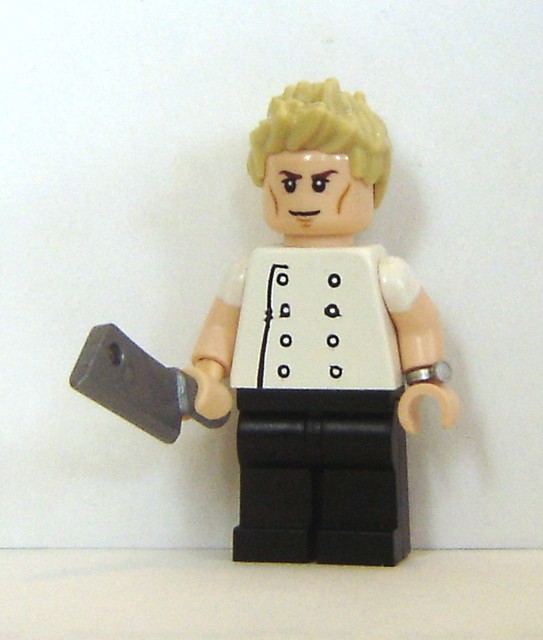This detailed, descriptive caption captures the elements from each voice description to create a cohesive portrayal:

In the center of the image stands a Lego figure resembling chef Gordon Ramsay. The character, with a frowning expression and blonde hair, appears angry. It is dressed in a chef’s uniform, featuring a white coat with black round buttons and black pants. On its left wrist, there is a visible silver watch, while its right hand clutches a silver or gray meat cleaver. The scene includes no text, only a mixture of colors — white, black, gray, tan, and blonde. The Lego figure is positioned against a plain white wall or background and stands on a hard, white surface, possibly a countertop or table, indicating an indoor setting.